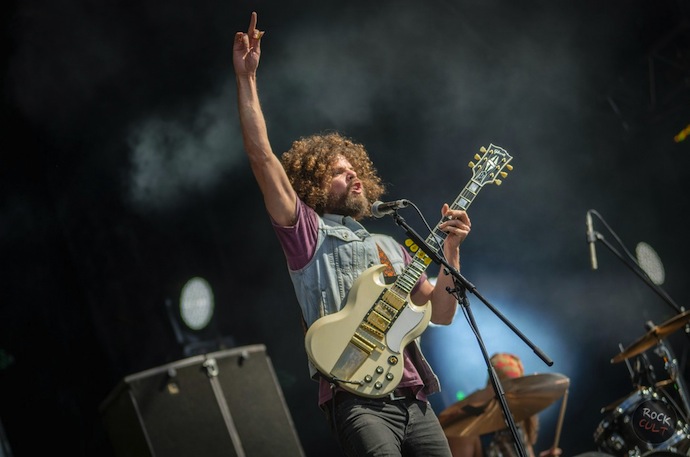This is a dynamic concert photograph predominantly showcasing an expressive guitarist. The horizontal, rectangular image is slightly angled to the left, providing an off-center view. The foreground features a white-skinned man with long, curly brown hair and a beard, resembling Sammy Hagar. He is captured mid-performance with his right arm raised high, flipping the middle finger, likely engaging the audience. The guitarist is dressed in a purple short-sleeved t-shirt under a light blue denim vest paired with dark gray jeans. 

He holds an off-white electric guitar with yellow accents, gripping the neck with his left hand. Behind him, the stage is set against a dark background with a hazy, smoke effect creating an atmospheric vibe. To the bottom right, parts of a black drum kit are visible. "Rock Cult" is emblazoned on one of the drums, with 'Rock' in white and 'Cult' in red letters on a black circular surface. The drummer is partially obscured, with only a drumstick and a metallic copper-colored high hat peeking into the frame. A large black amp and a small black lamp are positioned along the left edge of the image.